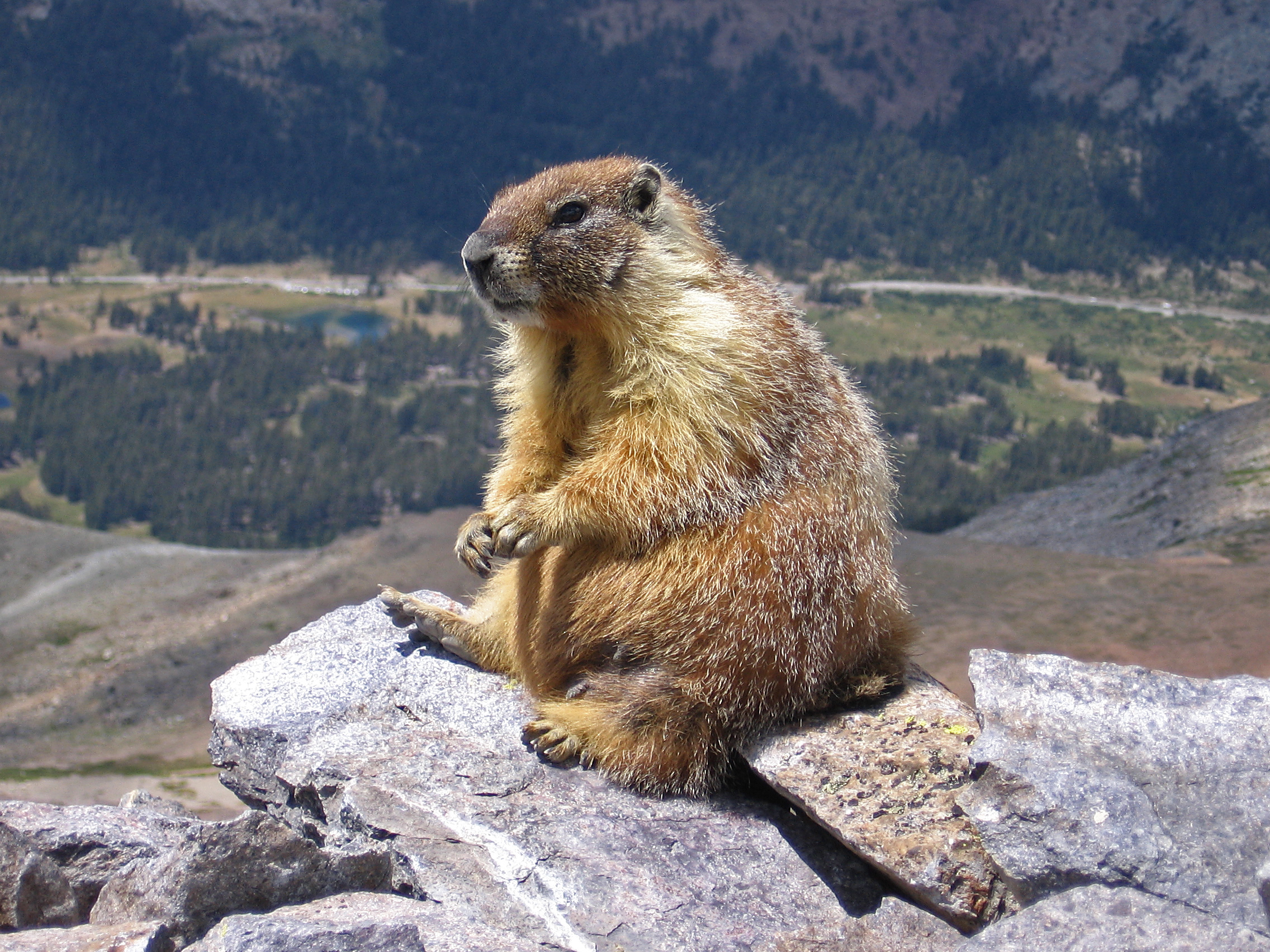A close-up photograph captures a chubby groundhog perched on a pile of rocks at the edge of a cliff overlooking a picturesque valley. The groundhog, with its brown and tan fur speckled with white tips, sits upright on its haunches, clasping its forepaws together. Its dark eyes and black nose stand out against its softly textured fur. The animal faces left in a profile view, seemingly surveying the valley below. 

In the distant background to the right, a small lake or pond glimmers, surrounded by a dense forest of trees. The valley stretches out below, flanked by hills that rise on either side, their slopes covered in verdant greenery. A winding road is visible at the base of the far hill, where a few cars are parked near the water's edge. The scene is devoid of buildings, emphasizing the untouched natural beauty of the landscape.